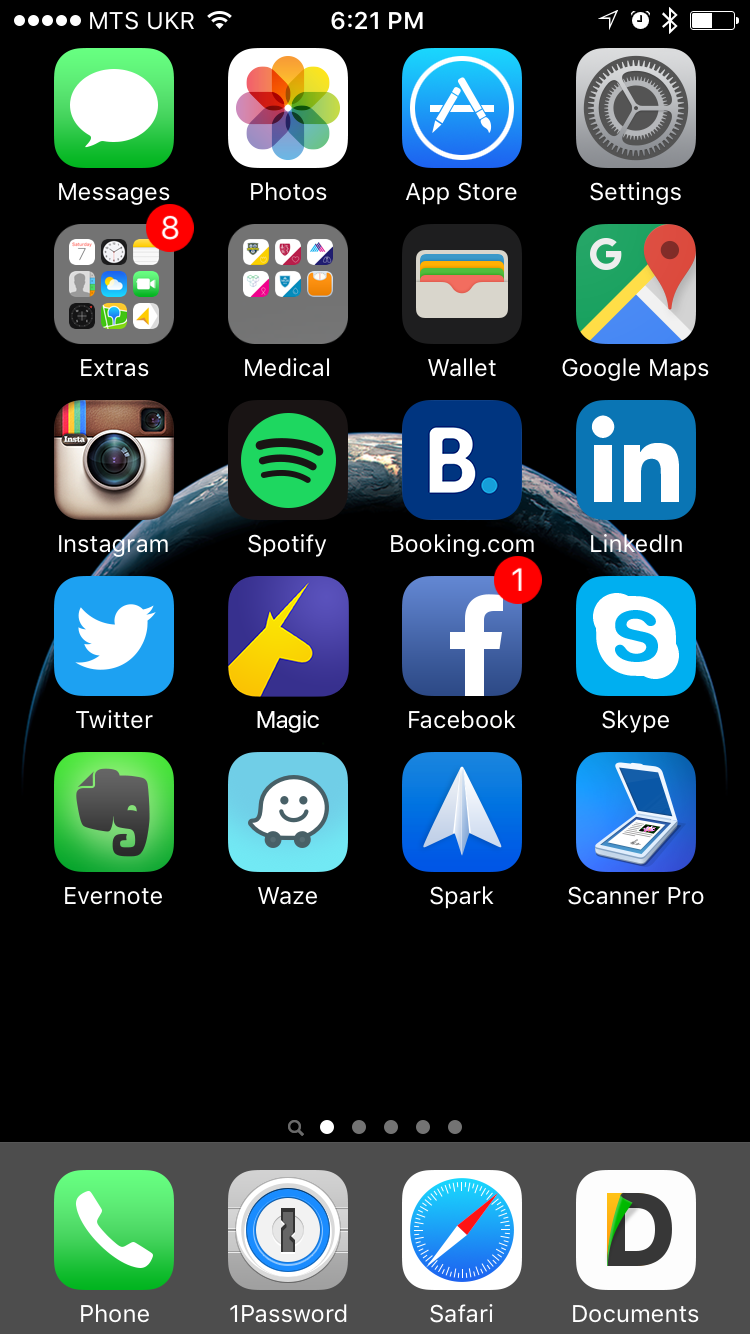**Detailed Caption:**

The phone screen displayed belongs to the "Websites" category and is depicted in its home screen mode. At the top of the screen, the status bar shows the label “MTSUKR,” alongside indicators for Wi-Fi and Bluetooth connectivity. The time displayed is 6:21 PM, and there's an icon indicating an active alarm. The battery level is approximately 50%.

The screen is organized with a series of icons arranged neatly. At the very bottom, the most frequently used applications are showcased, which include:
1. **Phone** - The default calling application.
2. **1Password** - A password management app.
3. **Safari** - The web browser.
4. **Documents** - An app for managing files.

Directly above the docked apps, the home screen exhibits a grid of additional apps:
1. **Messages** - A green icon with a white speech bubble.
2. **Photos** - Represented by a colorful flower.
3. **App Store** - A blue circle featuring a stylized 'A.'
4. **Settings** - Illustrated by a gear icon.
5. **Extras** - A folder containing 8 smaller, indistinguishable icons.
6. **Medical** - Another folder, holding 6 items.
7. **Wallet** - Depicted as a minimalist wallet with visible credit cards.
8. **Google Maps** - Identified by a map icon with a red location pin.
9. **Instagram** - Icon showing a simplified camera.
10. **Spotify** - Recognizable by its green circle with black sound waves.
11. **Booking.com** - Marked by a large 'B.'
12. **LinkedIn** - Displayed with the letters 'IN.'

Additionally, an array of social media and utility apps are also present including:
- **Twitter** - The blue bird icon.
- **Facebook** - The iconic 'F.'
- **Skype** - A blue 'S' within a bubble.
- **Evernote** - The green elephant.
- **Waze** - A smiling navigator logo.
- **Spark** - An email app depicted with a stylized paper airplane.
- **Scanner Pro** - Likely represented with an icon indicating document scanning functionality.

The arrangement and variety reflect a versatile use of the device, catering to communication, navigation, entertainment, and utility needs.